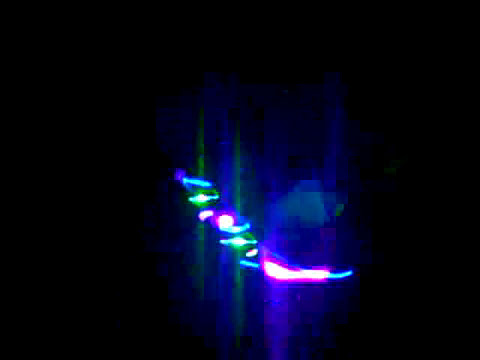The image in question is a low-quality, abstract piece with heavy pixelation and compression artifacts. The background is completely black, with the focal point being a glowing, smudged area in the center. This central portion features a chaotic mix of neon lights in various colors—blue, green, purple, and pink—arranged in shapes that resemble a leg and foot sticking out at an awkward angle. The neon lights appear to be poorly rendered, with their glow reflecting both above and below in a washed-out manner, further adding to the blurriness and degradation of the image quality. Additionally, a dark purple, oddly shaped circle occupies the center, surrounded by horizontal yellow section lines amidst the black backdrop. From the left and down towards the right, there are staggered neon lights, including some indistinct colors due to the heavy compression. The end result is an abstract, pixelated image marked by streaks of neon light amidst an overwhelmingly dark background, giving it an overall chaotic and indecipherable appearance.